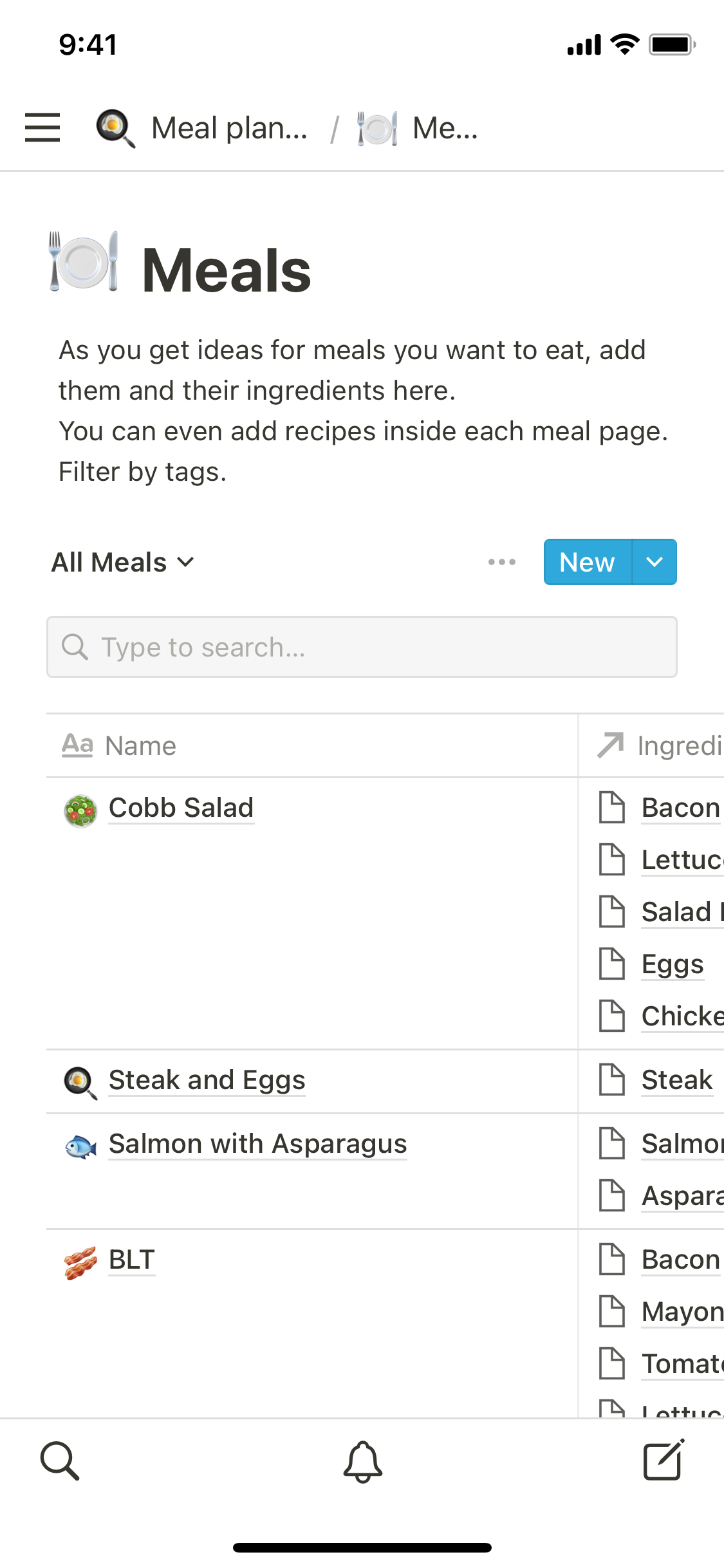**Detailed Caption:**

This image is a mobile screenshot of a meal planning app, captured at 9:41 AM. The battery icon on the top right indicates that the device is mostly charged. At the very top of the screen, the title "Meal Plan" is displayed along with a small icon of a frying pan containing a fried egg.

Below the title, there's a section labeled "Meals" with instructive text in black: "As you get ideas for meals you want to eat, add them and their ingredients here. You can even add recipes inside each meal page filtered by tags." Accompanying this text is a graphic of a white plate with a silver fork on the left and a silver knife on the right.

Underneath, there are two main segments: "All Meals" on the left and a blue "New" button on the right, designed for adding new meal entries. A search input bar is also present for quickly finding specific dishes.

Listed below are several meals with their respective ingredients and icons:
- **Cobb Salad**: Ingredients include bacon, lettuce, salad, eggs, and chicken. The dish is illustrated with a graphic of a salad.
- **Steak and Eggs**: Ingredients include steak, salmon, and asparagus. Visualized with an icon of a frying pan containing a fried egg.
- **Salmon with Asparagus**: Accompanied by an icon of a blue fish swimming to the left, with the main ingredients being salmon and asparagus.
- **BLT**: Ingredients listed are bacon, mayonnaise, tomato, and lettuce.

Each meal is presented with a small, relevant graphic, enhancing the visual appeal and user-friendliness of the app.